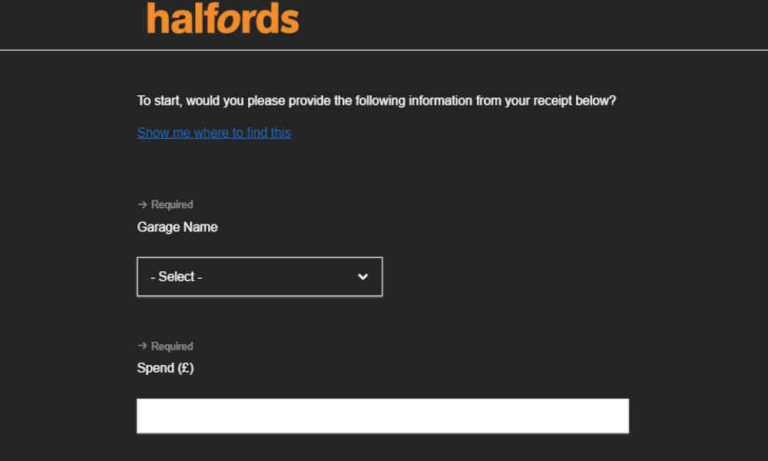Screenshot of a "HALFORDS" webpage displayed in night mode, with a black background and white text. At the top of the page, the name "HALFORDS" is prominently shown in large, orange lettering, situated in the upper middle-left section. Below and above this title, the entire page follows the night mode theme. 

The main body of the page prompts users with the phrase: "To start, would you like, please provide the following information for your receipt below." Beneath this text, there is a blue hyperlink labeled "show me where to find this."

Below this instruction, there are multiple form fields. The first field is labeled "Garage name" in white text with a drop-down menu that has "Select" as the default option. An arrow to the right allows users to reveal additional options from the menu. The second field is dedicated to spending details, marked as "required." It includes a bar to input the amount, which seems to be in Italian lira (though the currency symbol is not identified with certainty).

From the information provided, it appears this webpage is for processing receipt information, possibly related to garage or storage rentals. The simplicity and minimal content emphasize the form's purpose.